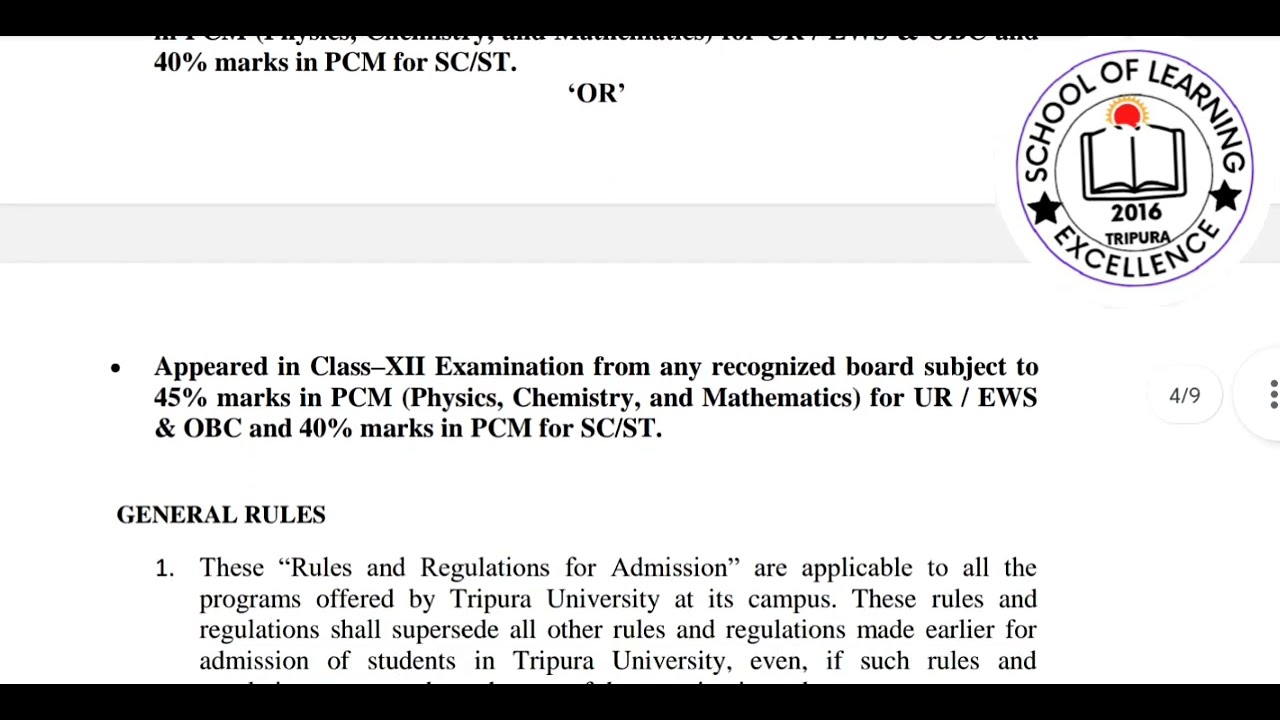The image shows a fragment of a document or slide from Tripura University. In the top right corner, there is a circular emblem featuring an open book in the center with the year "2016" and the word "Tripura" below the book. Surrounding the book is a sun diagram, and along the edge of the circle, the text reads "School of Learning Excellence." There are black stars flanking the words "School of Learning." The page is numbered 4 out of 9, indicated by a small white circle with the text "4/9" on the right side of the page, along with a grayish-blue bar running horizontally. The visible text on the page details eligibility criteria for class 12 examination results from any recognized board, requiring 45% marks in PCM (Physics, Chemistry, and Mathematics) for UR/EWS and OBC categories and 40% for SC/ST categories. Below this, general rules are listed, stating: "The rules and regulations for admission are applicable to all the programs offered by Tripura University at its campus. These rules and regulations shall supersede all other rules and regulations made earlier for the admission of students in Tripura University," where the text gets cut off.